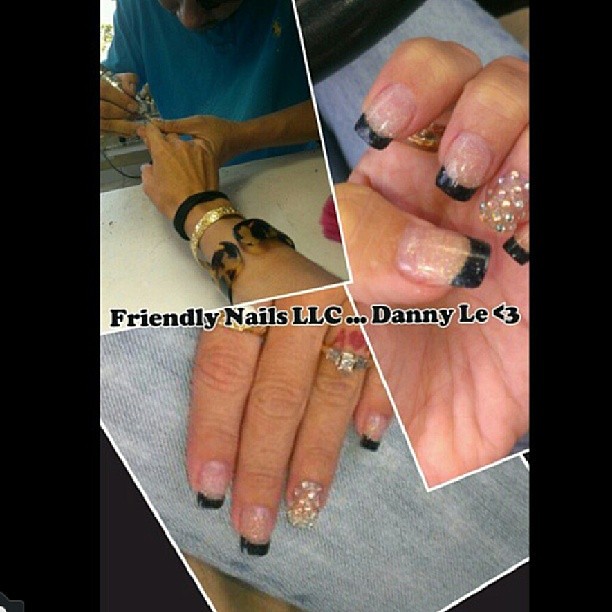The image is a collage within a central picture surrounded by black borders on the left and right sides. It captures various scenes in a nail salon, creating a vibrant tapestry of activity and designs. In the upper left corner, a man in a blue t-shirt is meticulously working on the nails of a client adorned with bracelets and bangles. Adjacent to this, on the right, there is an image of a lady’s fingers displaying an intricate nail design. Below these two images is another close-up of the same person's hand, showcasing finger rings on their index and ring fingers, highlighting their decorated nails. Centralized text reads "Friendly Nails, LLC, Danny L.E. <3," accentuating the friendly and professional atmosphere of the salon. The predominant colors in the image include black, white, green, blue, gray, gold, tan, and pink, and the setting appears to be indoors during the daytime. The entire collage fills the image, effectively presenting the essence and services of the nail salon.